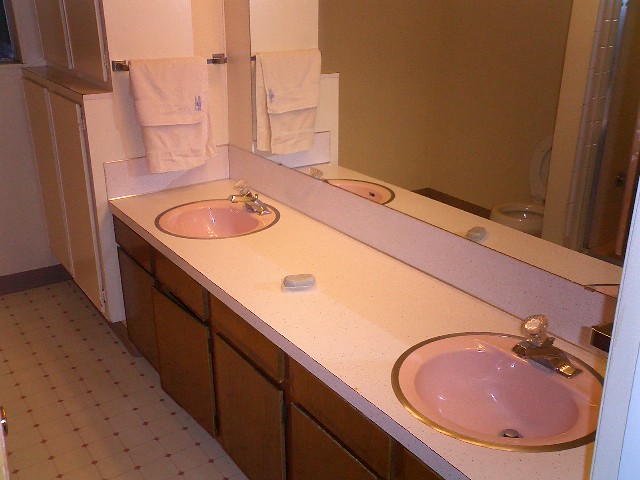The image depicts a vintage-style bathroom with a double vanity sink across the back wall towards the right. The two sinks are pink ceramic with a golden band around their circumferences and are oval-shaped, stretched out horizontally. Between the sinks is a large expanse of white formica work surface, which due to the slightly yellow lighting appears shadowy and speckled with light colors. Positioned centrally on the countertop, there seems to be a bar of soap. Above the vanity stretches a large wall mirror that reflects parts of the bathroom, including a white toilet. To the left of the sinks, there is a chrome towel bar holding some towels. Below the countertop are dark brown cabinetry units. The floor is covered with linoleum, featuring a geometric square grid pattern with thin lines and darker shapes at the intersections, suggesting a diamond motif. If you move past the double sink area, there appears to be a double-decker linen closet with center-opening doors, painted white. The overall retro aesthetic of the bathroom is accentuated by the materials and colors used, reflecting an older design style reminiscent of mid-to-late 20th century decor.